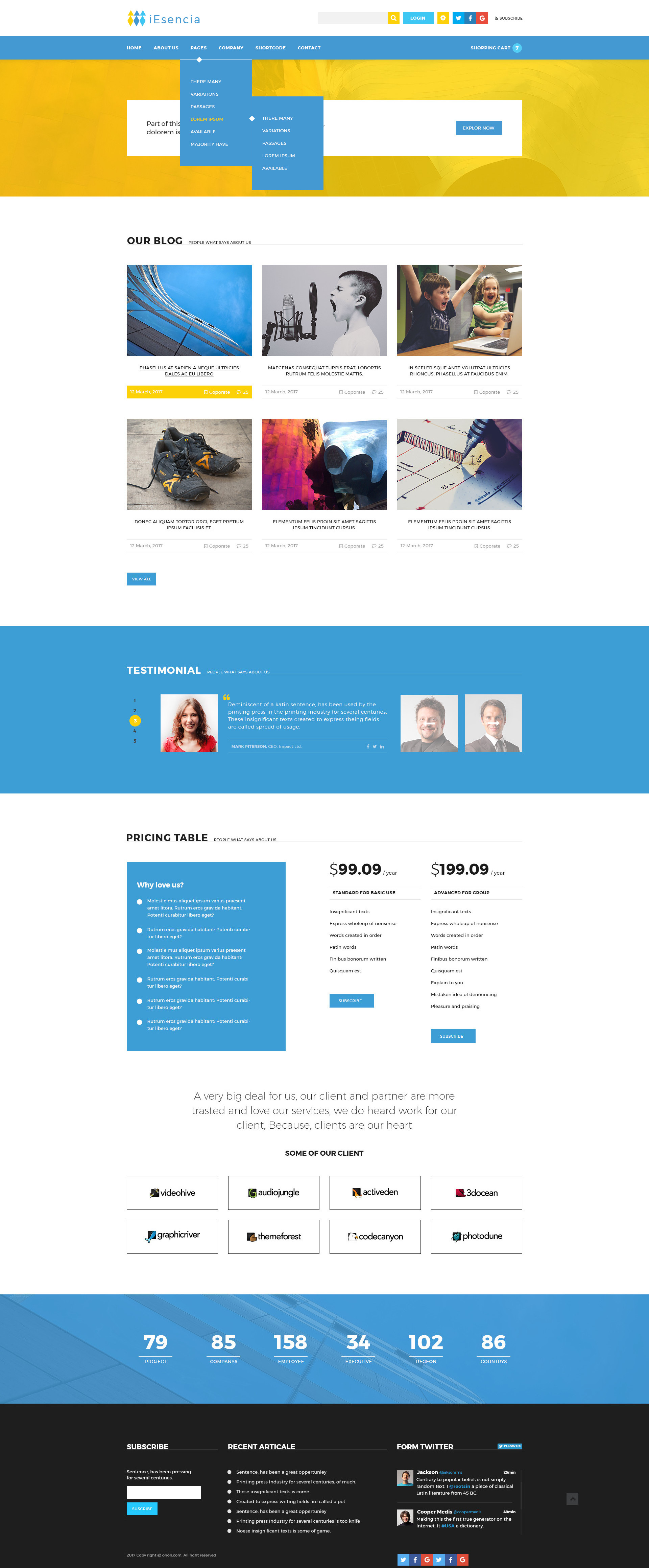This screenshot is from a webpage with a primarily white background. Although the screenshot is highly compressed and difficult to read, several elements are discernible.

At the top of the page, a white rectangular banner displays the website name "Ientia". Adjacent to the site name is an icon featuring blue and yellow colors, though its exact details are unclear. To the right of this banner, there is a search field, marked on its right end by a small yellow square with a white magnifying glass icon inside it. Alongside the search field, there are buttons resembling social media logos.

Below this banner, a blue bar stretches across the page, featuring text in white font. Within this bar, two blue drop-down menus are open, also displaying white text.

Directly beneath the blue bar, there is a prominent orange rectangle with a large white rectangle centered inside it.

Further down, the white background is led by a section header in black font that reads "Our Blog." Underneath, there are two rows containing a total of six images. The images depict various scenes: a roller coaster, a child speaking into a microphone, two children seated at a desk looking at a laptop, a boy raising his hands in excitement, a pair of dirty sneakers, an indistinguishable image, and someone writing in a notebook.

Below this blog section, another blue rectangle features images of people, though specific details about these images are not clear.